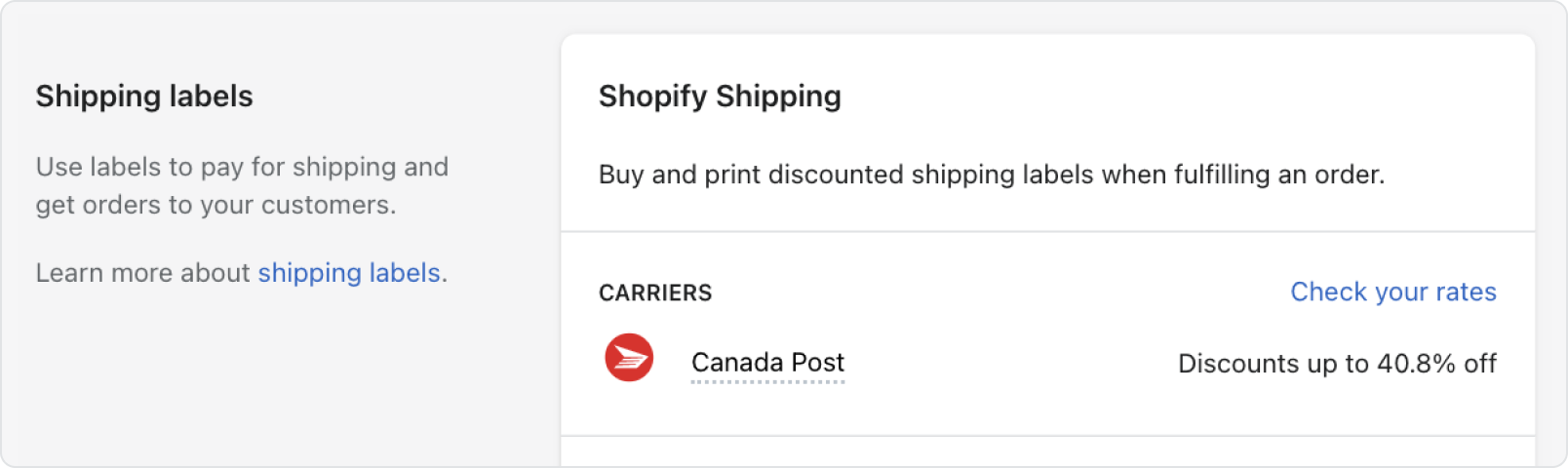This screenshot features a pop-up menu from a website showcasing options for shipping labels. The background of the pop-up is a very light gray rectangle. The content is divided into two sections: the left side featuring black text on the gray background and the right side containing a smaller white rectangle with additional text.

On the left side, in bold black font, the heading reads "Shipping Labels." Directly below, in regular black font, it explains: "Use labels to pay for shipping and get orders to your customers." Additionally, there is a clickable link with blue text that says "Learn more about shipping labels," which likely redirects to more information.

The right section contains a smaller white rectangle. At the top, in bold black font, it reads "Shopify Shipping." Below, in regular black font, it states: "Buy and print discounted shipping labels when fulfilling an order." A black horizontal line separates this content from the information below. Under the black line, the section begins with the heading "Carriers" in regular black font. An icon of a red circle with a white book follows, labeled "Canada Post" in black font, underlined with a dotted line. To the right of the icon, it notes: "Check your rates, discounts up to 40.8% off" in bold black font.